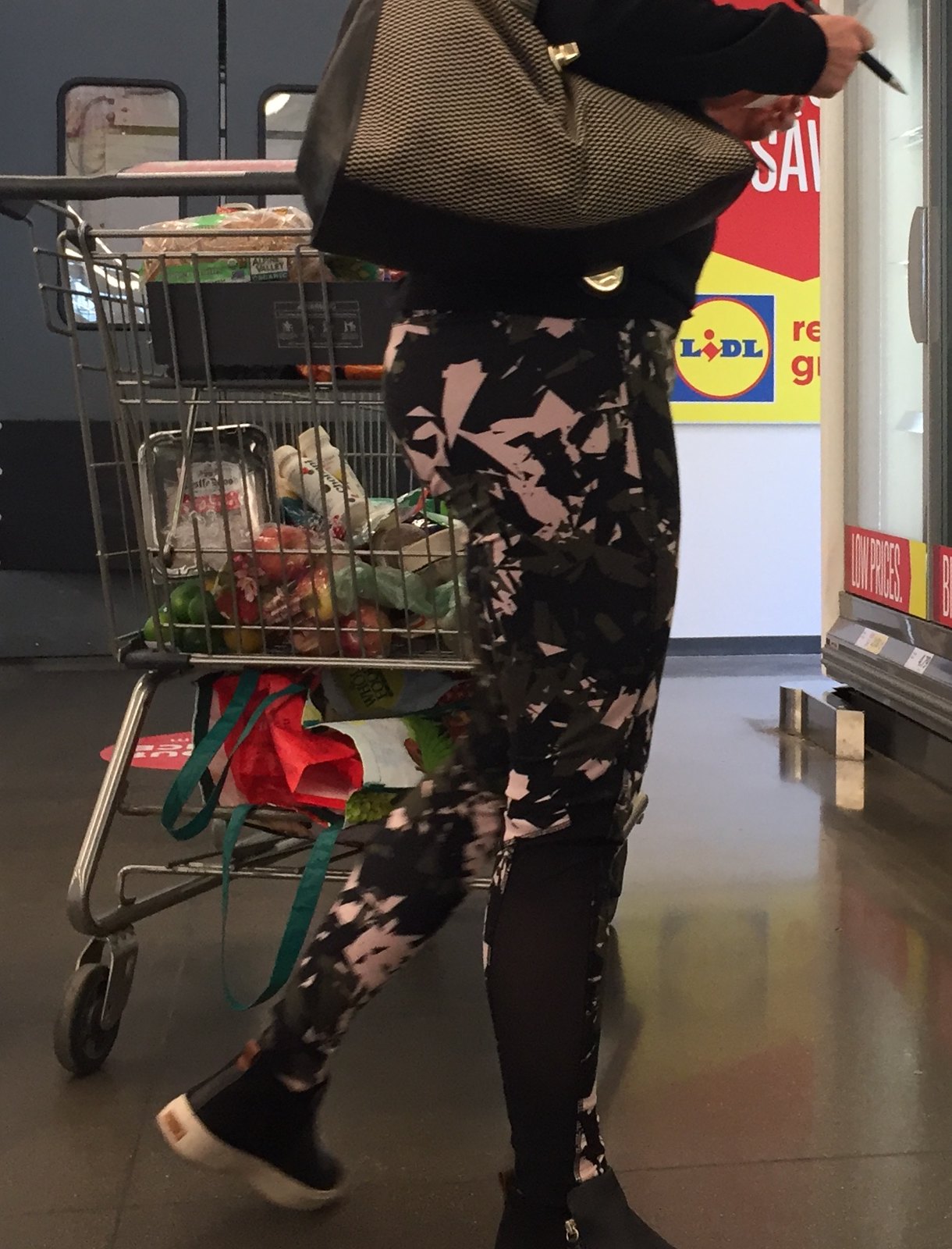This photograph captures a woman shopping in a Lidl grocery store from a low, strange angle, roughly around knee height. The image shows the lady wearing tight-fitting, geometric-patterned leggings in shades of black, pink, and possibly army green, paired with black high-top sneakers. You can see her legs, feet, and the lower portion of her body, including her black purse slung over her shoulder. She appears to be turning away from her shopping cart, likely reaching into a refrigerated case on the side. The shiny floor beneath her is a mix of gray and brown tiles.

Her shopping cart, metallic and silver, contains various groceries such as green and red peppers, foil pans, a loaf of bread, and other produce. The bottom rack holds a red reusable bag with green handles, suggesting she brought her own bags for shopping. In the background, a wall poster stands out with the word "SAVE" and Lidl's logo, a blue square on a yellow background. The overall scene is set against a white wall, adding to the clinical yet bustling atmosphere of the grocery store.